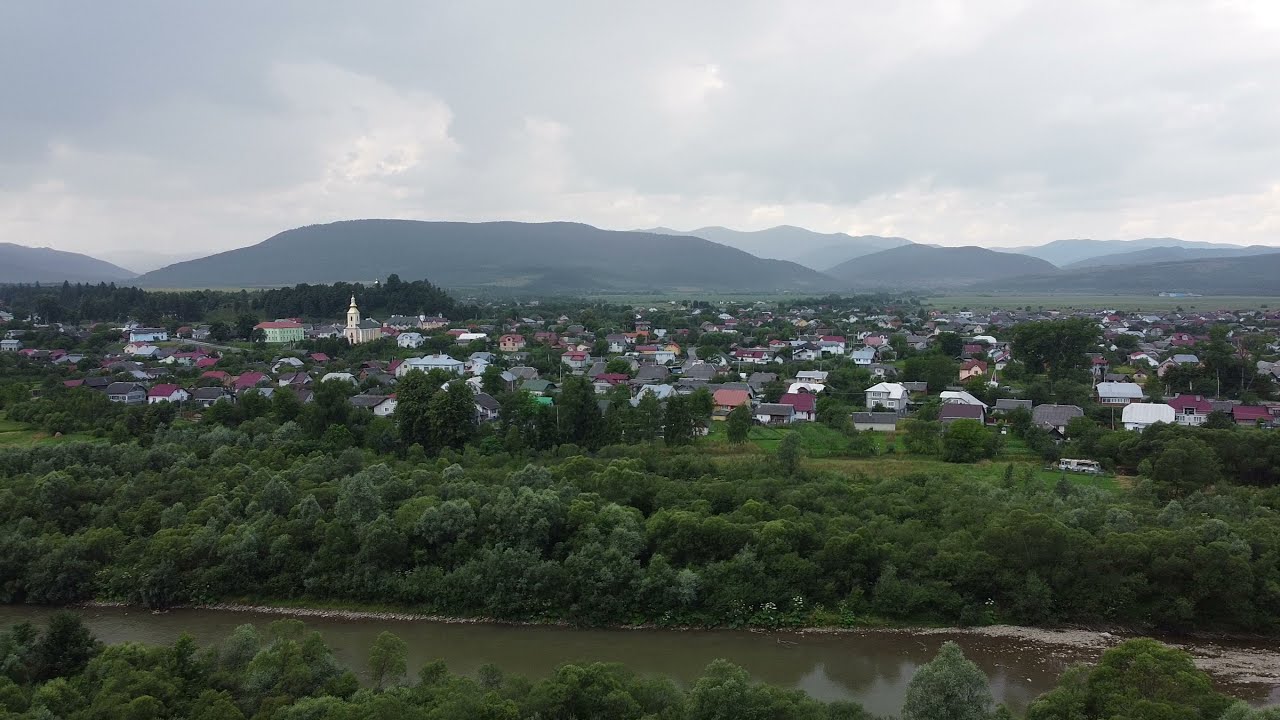This aerial drone photograph captures a scenic landscape in a horizontal, wide-angled view. At the very bottom of the image, a dark, green, murky river flows from left to right, bordered by a dense strip of trees. Above the river, a thick expanse of lush, green bushes and trees stretches horizontally, occupying about 15% of the image. Beyond this forested area lies a small town, with a variety of houses featuring roofs in shades of gray, white, red, and orange. Notably, on the middle left side of the town, there is a prominent white church with a tall tower or steeple. In the distant background, a series of low, dark mountains rise, partially obscured by a foggy haze. The sky above these mountains is filled with gray and white clouds, enhancing the overall atmospheric mood of the scene.